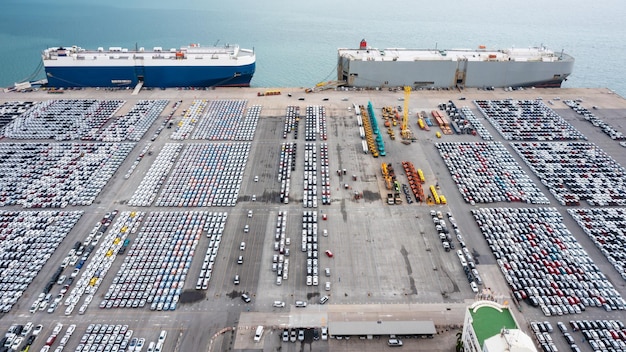This aerial photograph captures a bustling outdoor shipyard adjacent to a large, still body of water, possibly an ocean or gulf, with a seamlessly clear blue sky blending into the horizon. Dominating the scene are two massive docked cargo ships: the one on the left features a white top and blue bottom, while the one on the right appears predominantly gray or off-white with a distinctive red square peg visible. In the foreground sprawls an extensive parking lot teeming with rows upon rows of vehicles, numbering in the hundreds or more. Interspersed among the vehicles are trucks and various loading equipment, indicative of the shipyard's active operations. Several buildings housing supplies and materials for loading onto the ships are also visible, emphasizing the organized yet industrious nature of the port. No people are discernible in this expansive and meticulously detailed setting.